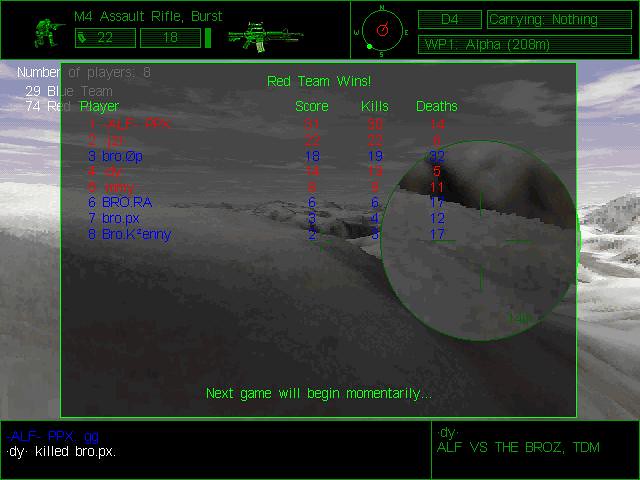The image appears to be a pixelated screen capture from a late 90s or early 2000s military-themed PC video game. The screen features a green HUD with a prominent "Red Team Wins" message in green font at the center, indicating the end of a multiplayer match. Below this, detailed statistics for the players are displayed, including the score, number of kills, and number of deaths, separated by team colors—red and blue. The bottom of the screen announces, "Next game will begin momentarily." On the upper left side, there is information about the M4 assault rifle set to burst mode, complete with an image of the rifle and ammunition details—numbers 22 and 18 are visible in green square boxes. Also on the left, an image of a soldier crouching, likely indicating the player's stance, accompanies these details. Additional text includes various player actions and game states in both white and blue fonts, such as "dy killed bro.px dot" and "elf-ppx."